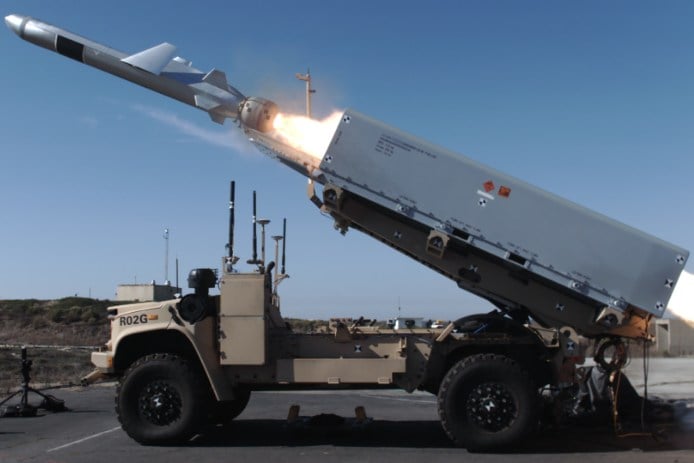This detailed image depicts a heavy-duty, military-grade wheeled vehicle situated on a paved surface, likely within a military base or near an airport. Central to the scene is a truck with no visible driver's cab, indicating it might be remotely controlled. On this truck is an elevated truck bed, akin to a dump truck mechanism, but instead of typical cargo, it houses a square, rectangular missile canister. The canister is pivoted upward at an approximate 20 to 30-degree angle for launching purposes.

Emerging from the canister is a rocket-powered missile, characterized by folded wings situated mid-body, suggesting it's mid-launch with its wings soon to deploy. The missile is captured just as it clears the canister, trailing visible fiery exhaust. The backdrop includes a clear blue sky devoid of clouds, a rocky hillside adorned with patches of grass and bushes, and a dirt road. Scattered in the distance are silver container boxes and buildings, adding to the militaristic ambiance of the image. The overall scene is bathed in sunlight coming from the upper left, enhancing the vividness of the missile's fiery exhaust as it embarks on its mission.